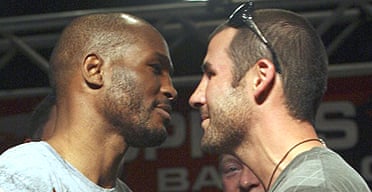This grainy close-up photograph captures a tense moment between two men standing face-to-face, their noses mere inches apart. The man on the left has dark skin, closely cropped hair, and a short beard. He wears a light blue or gray crewneck t-shirt and a black necklace, with sunglasses resting on top of his head. His expression is a mix of slight contempt and a faint smile. The man on the right, who has fair skin, equally short brown hair, and a matching stubble beard, is dressed in a gray t-shirt adorned with a light gray diamond pattern. His sunglasses are also perched atop his head. In the background, partially obscured behind both men, are two other individuals – a third man peering from beneath the right-hand man's neck and someone else's cropped hair behind the left-hand man's neck. Additionally, a red sign with unreadable white text and a corrugated metal beam are visible, suggesting an urban or event setting. The scene is evocative of a pre-fight stare-down, filled with palpable tension and the hint of a forthcoming confrontation.